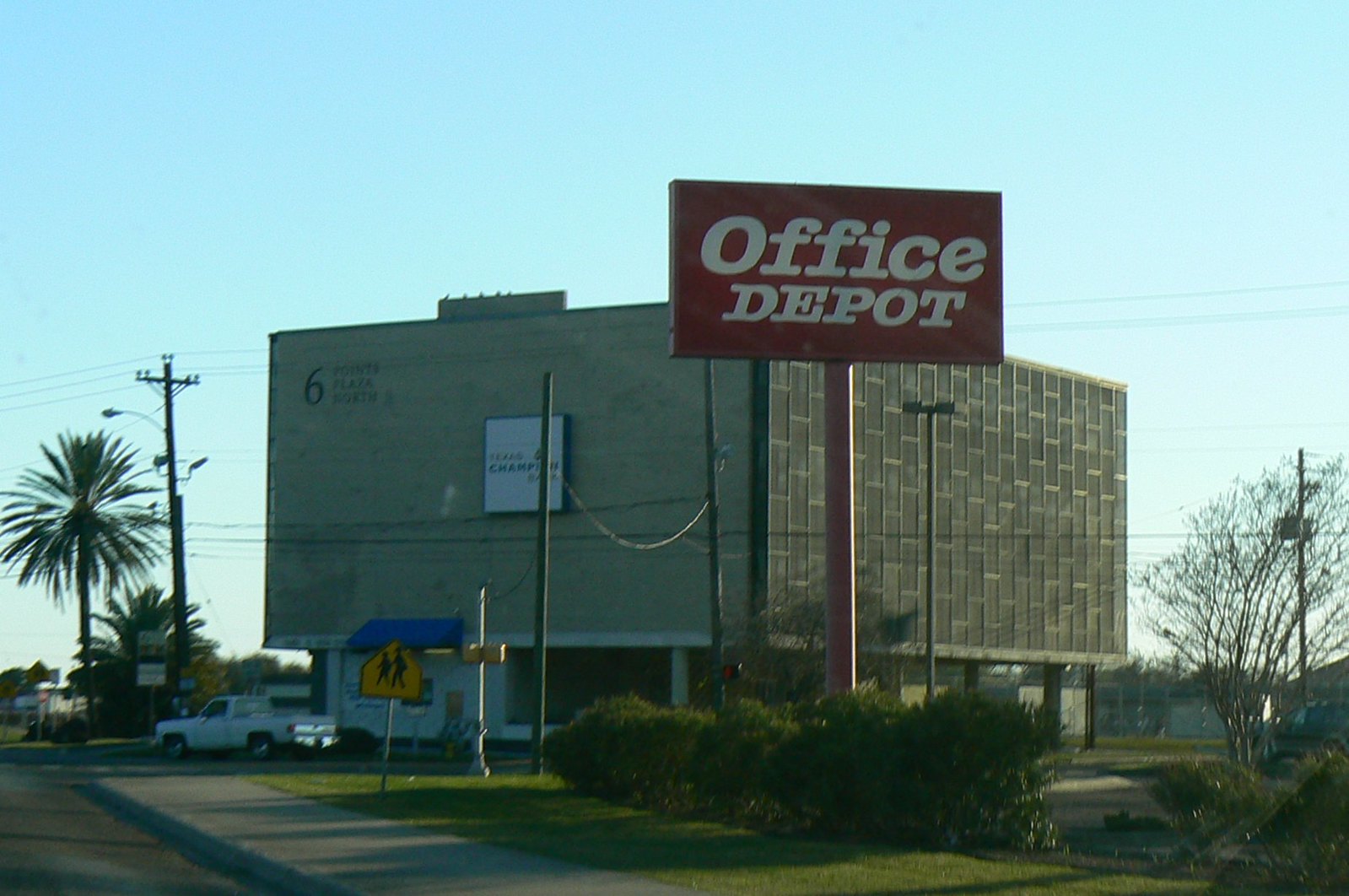In this image, we are taken to a tropical area that is transitioning out of winter. On the left side of the frame, a tall pine tree stands, while a more typical deciduous tree is situated on the right. Between them, there's a school zone sign equipped with a light, indicating caution nearby. Dominating the center background is a large, red Office Depot sign, suggesting the presence of the store in the vicinity. Behind the sign is a building labeled "Building Six," characterized by numerous windows on the right side and a blank wall on the left.

The scene is bathed in the soft light of an early morning sunrise, with elongated shadows adding to this serene morning ambiance. Surrounding the Office Depot sign is an area overgrown with untrimmed shrubbery, offering a sense of natural disarray. In the background, power poles are faintly visible, a reminder of the area's infrastructure. The Office Depot sign, although intended to be illuminated, remains unlit at this early hour. The overall image captures the quiet, slightly untamed charm of the location as it wakes to a new day.